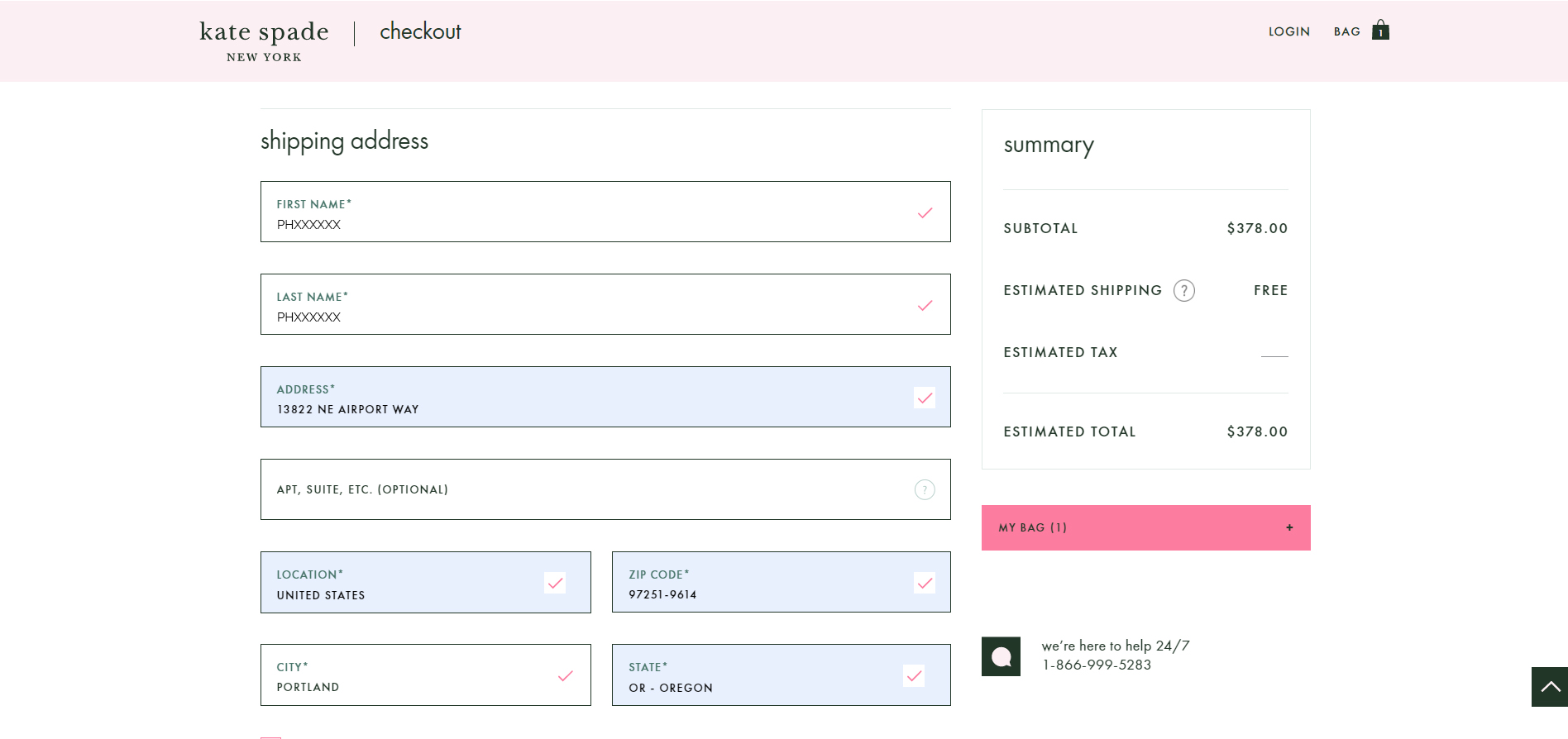This screenshot from the Kate Spade New York website depicts the checkout page. 

At the top, there's a pink navigation bar. On the left side of this bar, it reads "Kate Spade, New York" and "Checkout" in elegant fonts. On the right side, the navigation bar includes options to "Login" and view the "Bag," with a shopping bag icon symbolizing the latter; this icon has a number "1" inside it indicating one item in the cart.

Below this bar, the focus shifts to the "Shipping Address" section. Here, text fields are displayed for inputting personal information: "First Name" and "Last Name," both showing placeholder text "PHXXXXX.” The address field reads "13822 Northeast Airport Way" as a sample entry, followed by fields for "Apartment Suite, etc.," "Location" marked as "United States," "Zip Code" as "97251-9614," the "City" as "Portland," and the "State" as "Oregon."

On the right side of the screen, there is a summary box outlining the purchase details. This box breaks down the costs with a "Subtotal" of "$378," "Estimated Shipping" marked as "Free," and a blank for "Estimated Tax." The "Estimated Total" matches the subtotal of "$378."

Just beneath this, there is a horizontal pink line containing the text "My Bag" followed by the number "1," denoting the single item in the shopping bag, and a plus symbol on the far right. 

The overall design is clean and user-friendly, with key details prominently displayed to facilitate the checkout process.